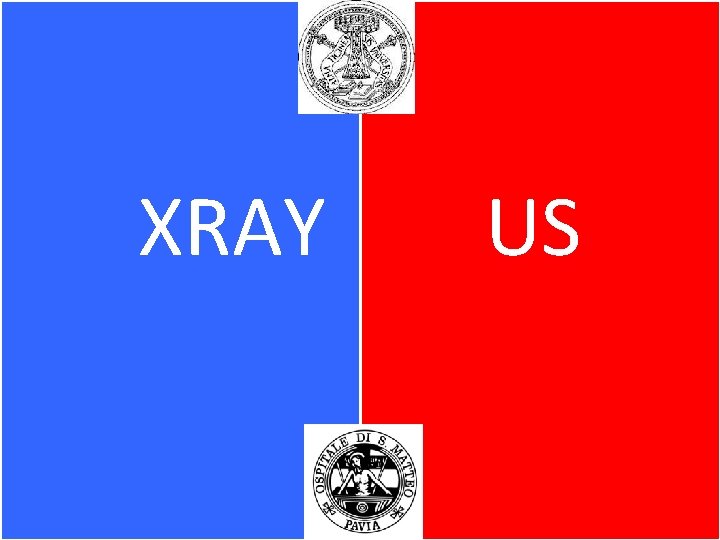The image is a horizontal rectangle divided into four sections. The left side features a vertically oriented blue rectangle with white, capitalized text that reads "X-RAY." The rectangle on the right mirrors this in size but is red, with the word "US" in white, capital letters in the center.

Dominating the middle portion of the top section is a white square containing a black, circular logo that consists of a circle with a cross in the middle and what appears to be a cone shape above it. 

At the very bottom, centered, is another white square housing a circular logo. This logo depicts a male figure, which some interpret as Jesus, with surrounding text that says "Optitel de Est Mato Paphir."

The predominant colors in the image are blue, red, white, and black, and the logos feature intricate designs and text, adding layers of detail to the overall composition. The two logos, located at the top and bottom, create a sense of symmetry and balance within the colorful rectangular halves.